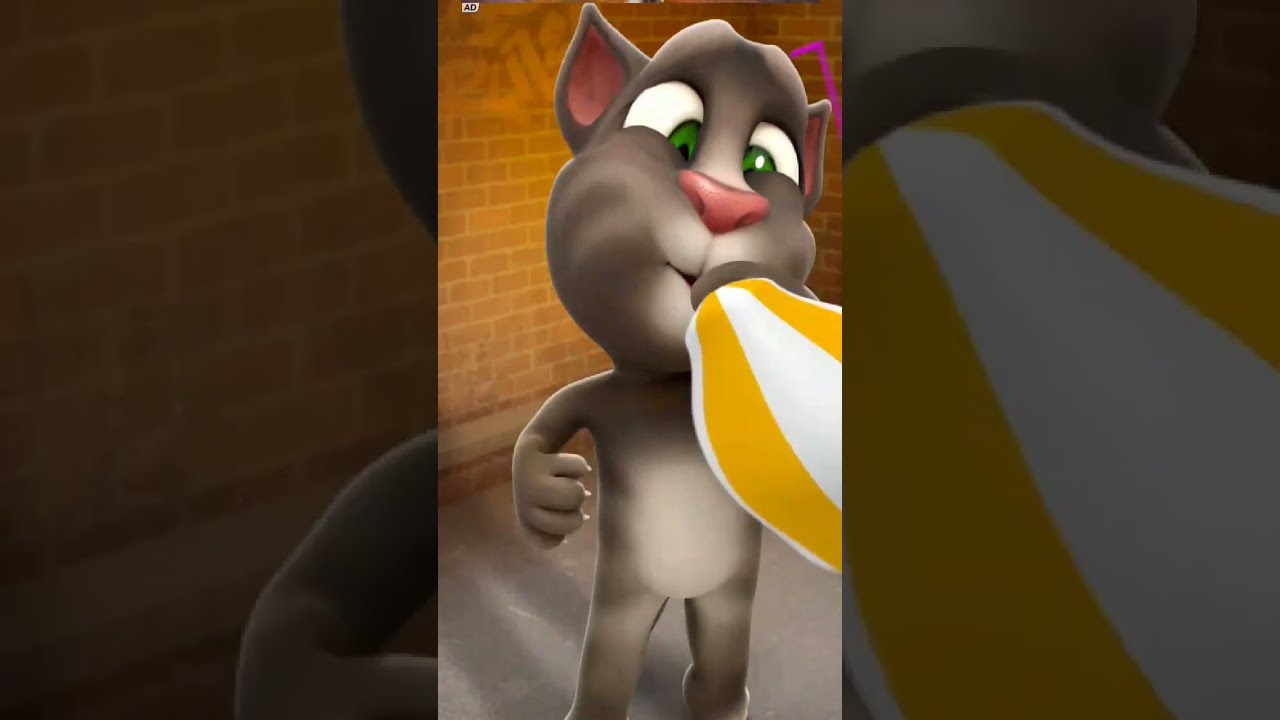The image depicts a computer-generated cartoon of a gray anthropomorphic cat with striking green eyes and a pink nose, set against a backdrop of a faded red brick wall with hints of graffiti in orange and hot pink lines. The cat is positioned in front of this wall, standing on a gray, cement-like floor. In its mouth, the cat holds a rounded object with white and yellow stripes, resembling a bottle. The lighting originates from the right, casting the cat's shadow to the left. The central focus of the image is confined within a vertical rectangle, where the cat appears cross-eyed, intently gazing at the striped object. Surrounding the central rectangle is a larger, zoomed-in version of the same scene, highlighting portions of the cat and the object it is holding.